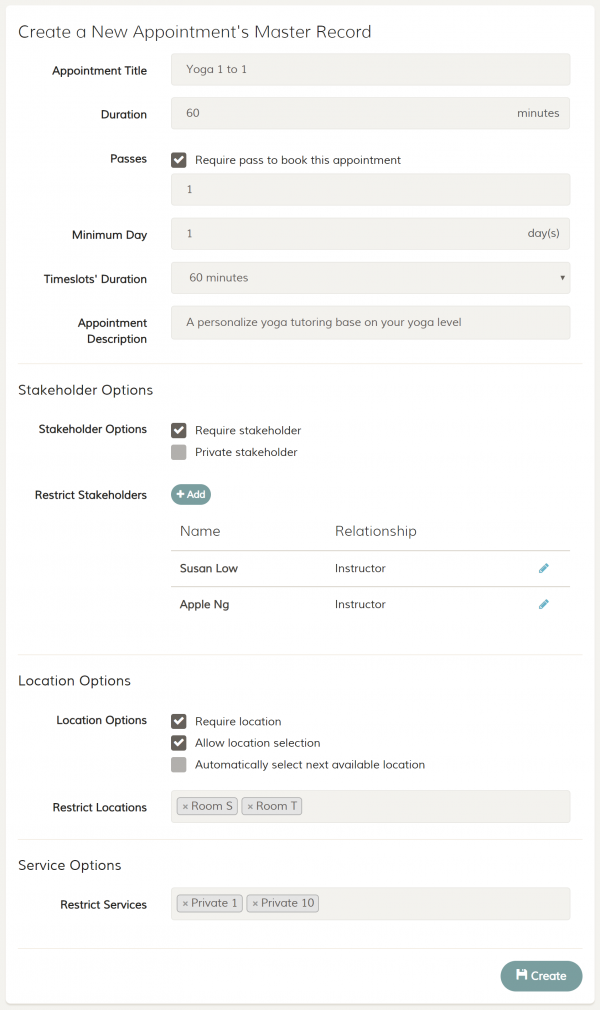This website screenshot features a gray border surrounding the entire image. At the top left corner, bold text reads "Create a New Appointments Master Record," with each significant word capitalized. Below, in a smaller, darker text, various input fields and options are displayed.

1. **Appointment Title:** "Yoga One-to-One"
2. **Duration:** "60 minutes"
3. **Pass Requirement:** A checkbox indicates that a pass is required to book this appointment.
4. **Minimum Days in Advance:** "1"
5. **Time Slot Selection:** Another field with a dropdown option specifies the duration of "60 minutes".
  
**Appointment Description:** "A personalized yoga tutoring based on your yoga level."

**Stakeholder Options:**
- Stakeholder requirement options are provided: "Require Stakeholder" is selected from the choices, which include "Private Stakeholder."
- Options to restrict stakeholders are mentioned.
  
A banner with white text shows fields for stakeholder information:
- **Name:** "Susan Law," **Relationship:** "Instructor"
- **Name:** "Apple NG," **Relationship:** "Instructor"

**Location Options:**
- "Require Location" and "Allow Location Selection" are selected.
- "Automatically Select Next Available Location" and "Restrict Your Locations" are also options. The selected rooms are listed as "Room S" and "Room T."

**Service Options:**
- "Restrict Services" is selected, with options such as "Private One" and "Private 10."

At the bottom of the form, there is a button labeled "Create."